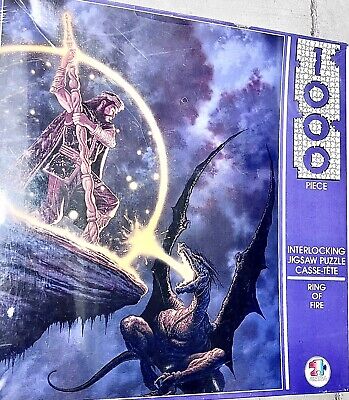This image showcases the front cover of a thousand-piece jigsaw puzzle set. The cover features a dramatic scene set against a cloudy purplish-blue background with hints of dark blue. To the far right, in white lettering, it says "Interlocking Jigsaw Puzzle" along with "Kasei Tatei Ring of Fire." At the top, prominently displayed, is the number "1000" indicating the piece count.

The central image depicts a warrior standing resolute on a dark blue cliffside. Clad in brown pants, a brown vest jacket, a cape, and a headband, the warrior plunges a staff into the ground. From this staff, a brilliant white light emanates, forming an orb of protection around him. Hovering near the warrior, a formidable black dragon expels a stream of fire from its mouth, which clashes against the protective orb. The intense contrast between the fiery assault and the magical shield forms a captivating and dynamic scene, set under the ethereal, stormy sky.